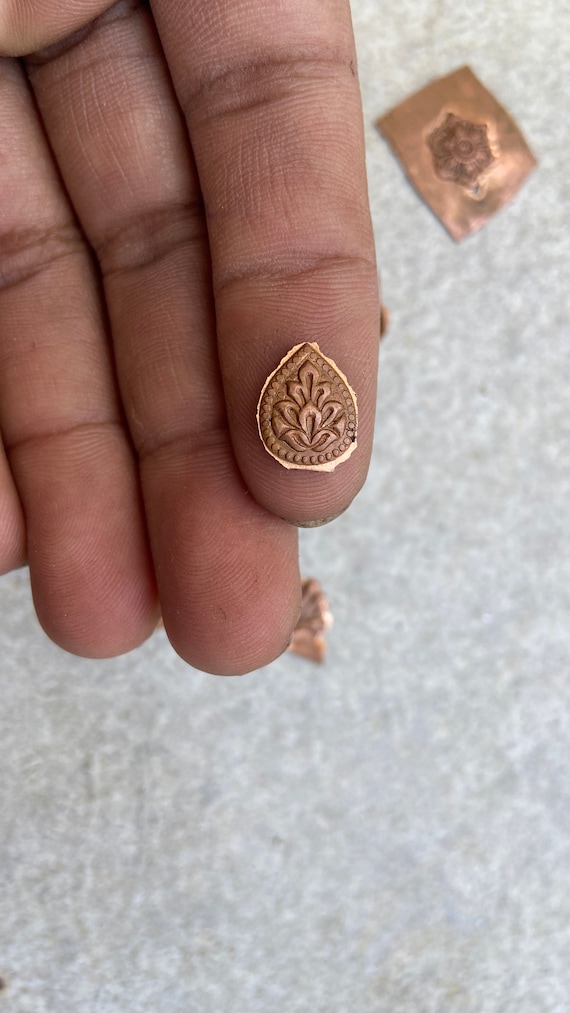This is a vertically oriented, realistic photo showcasing a close-up of a medium brown-skinned hand with visible creases and short nails, set against a whitish-gray background. The palm is facing up, and three fingers – the index, middle, and third finger – are prominently displayed, with a hint of the fourth finger visible. The hand appears dry, with the crevices colored, perhaps by dirt.

The index finger is holding a small, bronze-colored, tear-shaped medallion with intricate, lotus-like floral designs and a dotted border, giving the impression of a handmade piece due to its rough edges. A similar medallion lies on the gray background and another peeks out under the middle finger. The background's color and texture match the bronze aesthetic of the medallions, creating a cohesive visual theme.